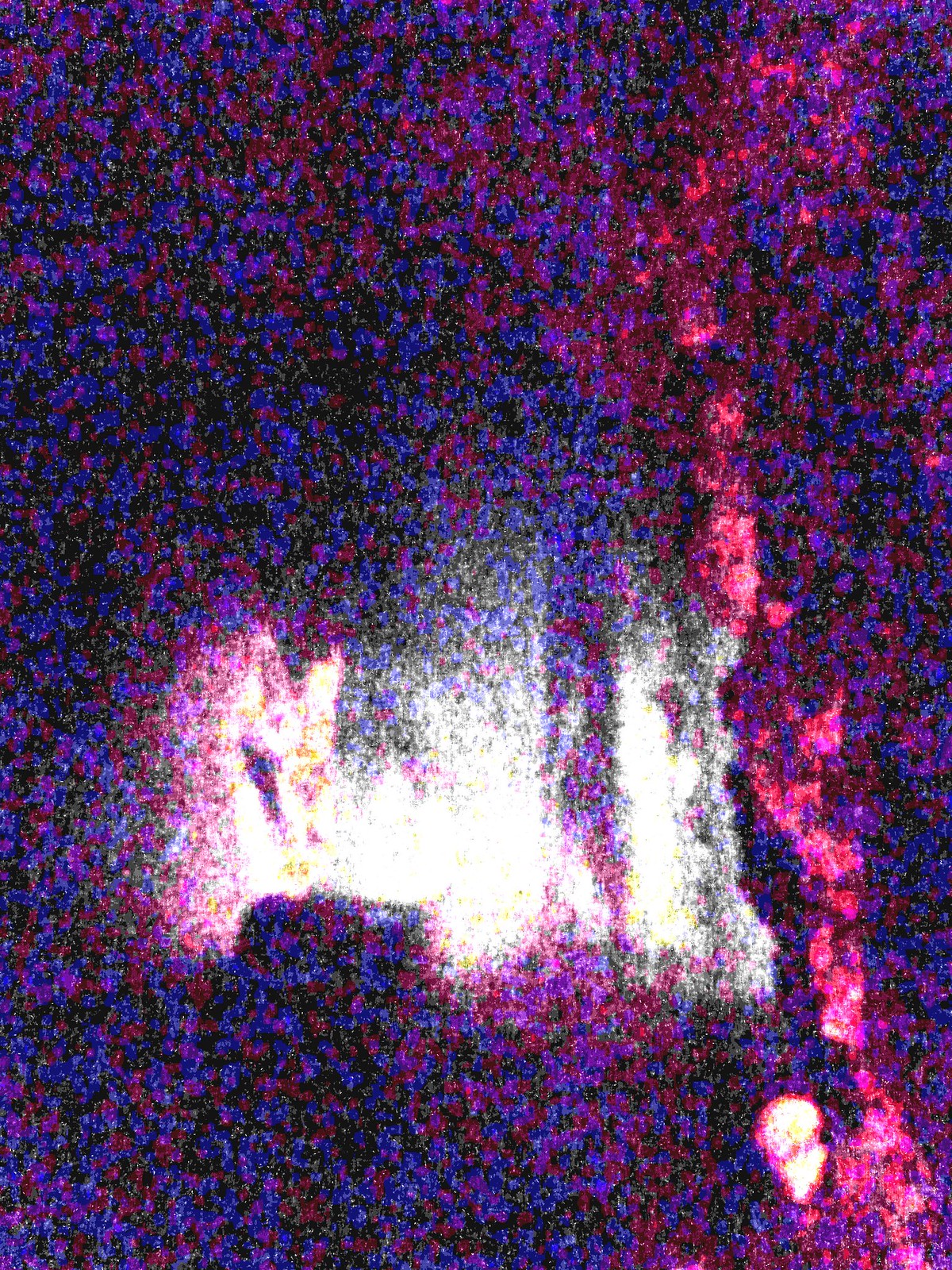This image is a highly pixelated, low-quality photograph dominated by specks of various colors. The predominant hues are black, red, and blue, mixed with occasional purple and orange specks. In the center, a vague white area stands out against the chaotic background, potentially resembling figures, possibly a band performing, evoking the ambiance of a concert. This white mass, coupled with the surrounding colorful speckles, creates a scene that appears dynamic but remains undefined. Towards the bottom right corner, there's a small, round white spot that could be interpreted as a face amidst the vibrant colors. A distinct, long red streak stretches vertically through the image, adding to the abstract nature of the snapshot. Overall, the photo is an enigmatic blend of dark and bright hues, providing a rough, almost surreal impression of what might be a lively moment captured with poor clarity.